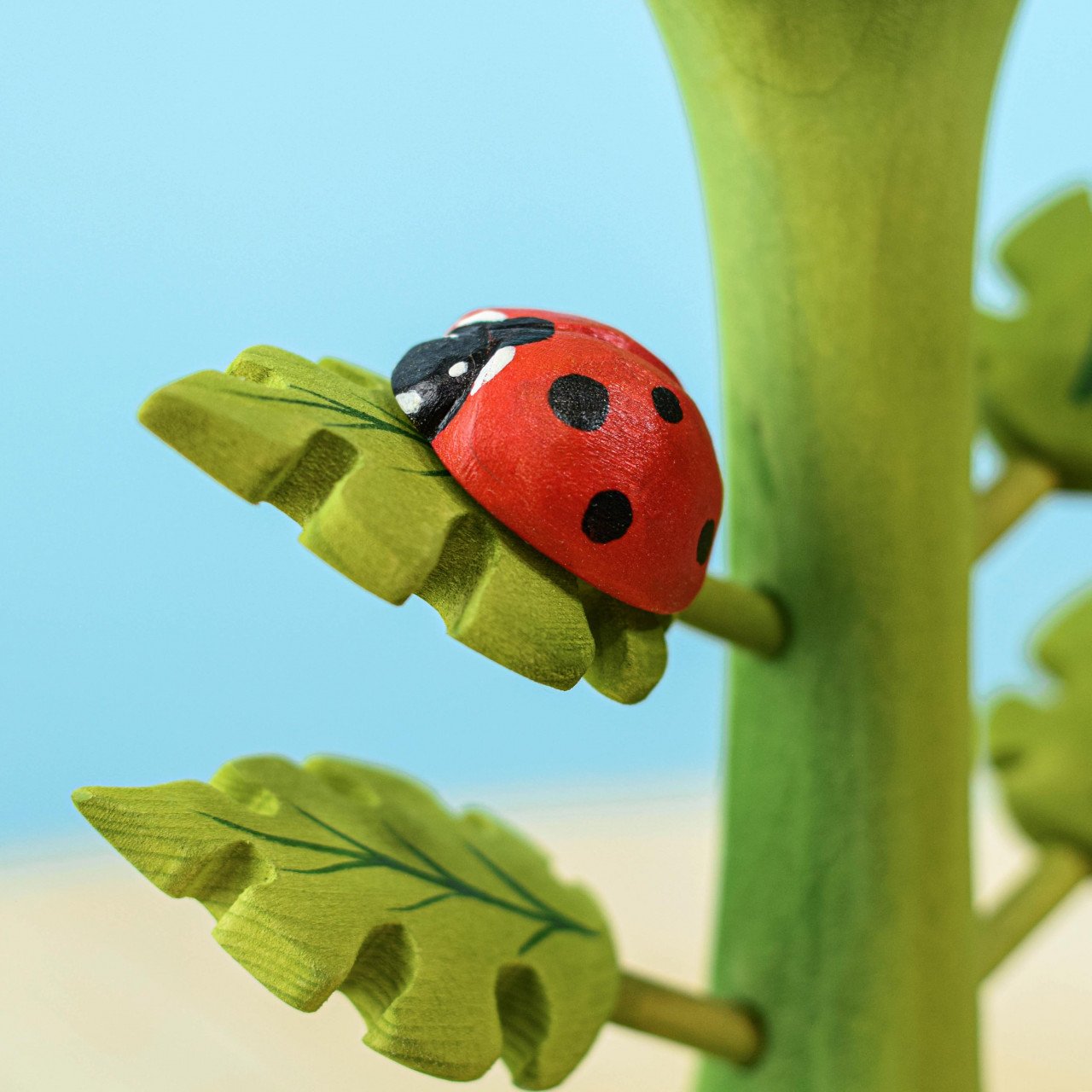This image features a close-up, professional-quality photo of a wooden piece of art meticulously designed to resemble a leafy plant or perhaps a vegetable stalk. The central structure is a vibrant green stem adorned with individually crafted branches and veins, highlighted with darker green hues to enhance the textural details. Perched on the top left leaf is a strikingly vivid ladybird, or ladybug, with a rich red body adorned with distinct black spots and a black head, showcasing true-to-life coloring. The background is artistically blurred, featuring a soft gradient of light blue representing the sky and a sandy beige at the bottom, possibly indicating the ground. The wooden texture of the leaves, complete with visible wood grain and striations, adds to the naturalistic and handcrafted charm of the artwork. This detailed depiction suggests that the piece may have been created as a home art project, capturing nature's delicate beauty in a tactile, painted wooden form.